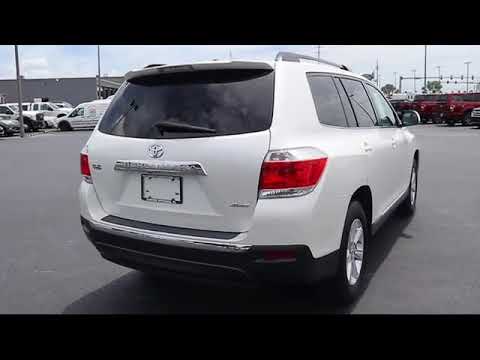This photograph captures the rear three-quarters view of a white Toyota station wagon parked in a parking lot. The vehicle, with dark-tinted windows including the rear windshield that features a wiper, prominently displays the Toyota emblem beneath the back window. Equipped with a dark gray bumper and red taillights, the station wagon is outfitted with a luggage rack on top, outlined by several rails. The car, parked at a slight angle, reveals two of its four doors and wheels. 

The parking lot is surfaced with gray concrete and contains multiple vehicles, including other white vans to the left and a couple of red trucks or Jeeps to the right. The background features an industrial concrete building and a light blue sky above, further indicating that this could be a city scene. On the right side, traffic lights are visible, reinforcing the urban setting. The image itself is framed with a thin black header and footer, with no borders on the sides.